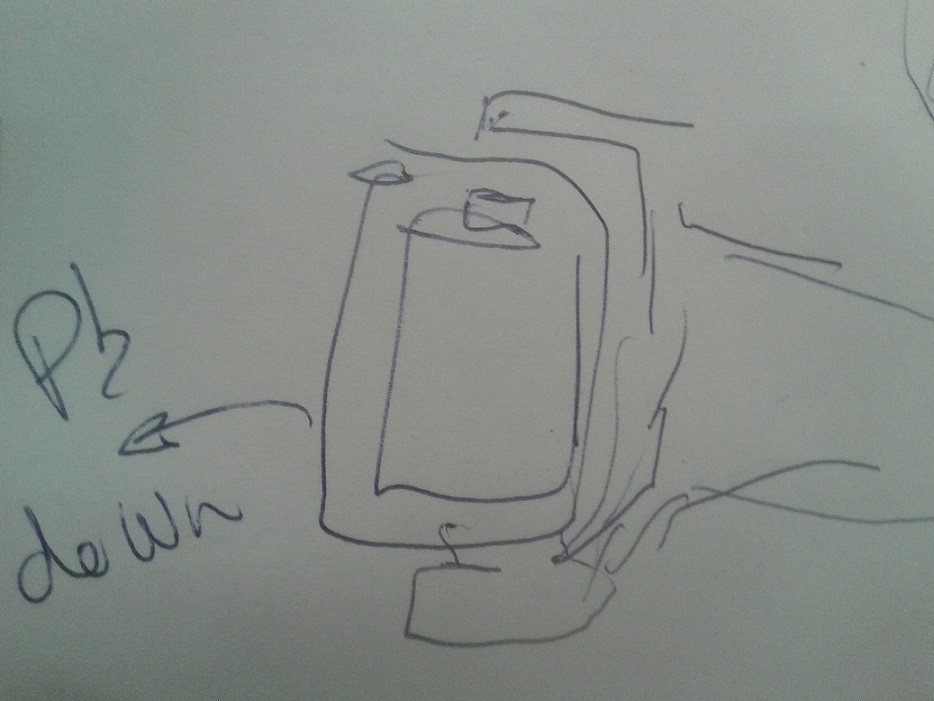This detailed pen sketch, created in black ink, features a rudimentary illustration of a pipe fitting. Central to the sketch is the pipe, depicted with an opening and intricate details capturing its structure. An arrow near the pipe points to the left, accompanied by handwritten text to its left. The text displays a capital letter 'P' followed by a lowercase 'b' above the arrow, and the word "down" positioned directly below it. Additionally, the sketch includes an element with a square hole, seemingly part of a framed structure linked by a rod. The overall drawing is rough and appears to be a quick conceptual diagram or technical doodle, highlighting the basic components and their directional orientation.